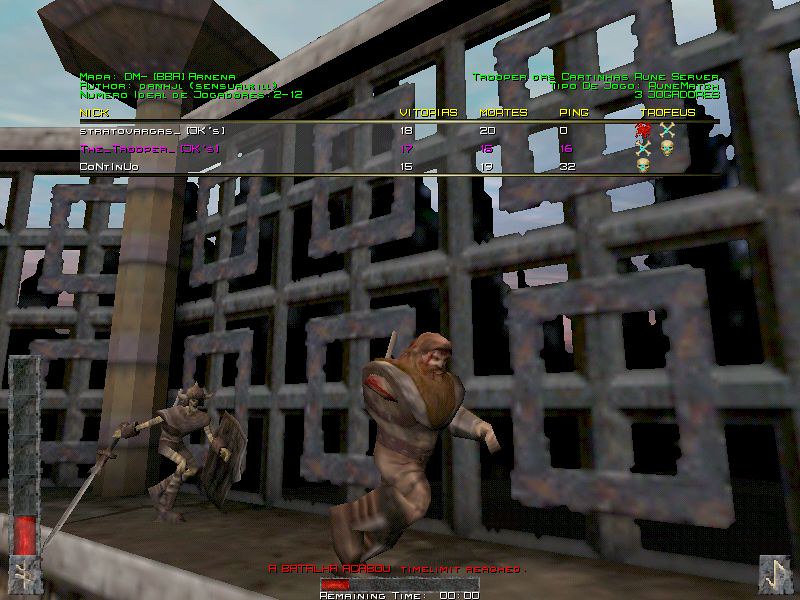The image is a detailed screenshot from a video game, featuring two central characters running along a mottled green and brown path. In the foreground, a man with long brown hair, a long brown beard, and thick fur clothing is missing his right arm and holds his left arm out in front. He is chased by a skeletal warrior a few steps behind, equipped with a horned helmet, a large sword in one hand, and a shield in the other. The background showcases a metal fence with square patterns. Text overlaying the image includes various game-related information: in green letters at the top are "MAPPA DM BBR ARENA AUTHOR DAN HJL NUMERO IDEAL DE JAGRADORES," while the bottom part of the screen displays the phrase "Batrala Akrabu time limit" in red letters and a progress bar indicating "remaining time: 00:00." Additional text below the progress bar reads "VITORIAS," "MORTS," "PENG," and "TROPHEUS."